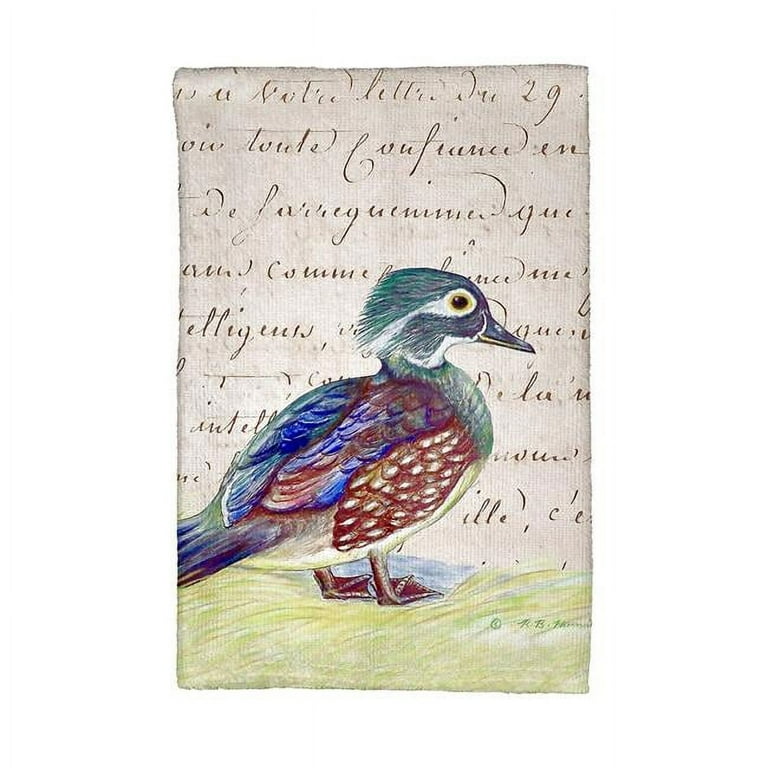This is a photograph of a handmade piece of art, depicting a colorful duck standing on a nest-like area. The art is set within a rectangular frame measuring approximately five inches high and four inches wide, with faint vertical lines forming a border on either side. The top three-fourths of the background features a light brown hue overlaid with cursive words in dark brown, which are difficult to read. 

The focus of the artwork is the duck, centrally positioned and facing right. Its head and back are adorned with various shades of bluish-green and purple feathers, with distinct yellow circles around its black eyes. The beak is black with a yellow line separating the upper and lower parts. The duck's chest has a green color, while its front throat is white. The belly is a blend of white and greenish tones, and the wings exhibit a combination of brown adorned with white specks, and blue highlights. The tail feathers are a mix of blue, gray, and red, and the webbed feet are a reddish-orange color. 

The duck is illustrated standing in a slightly gray area surrounded by green grass. In the lower right corner of the drawing, there is a signature reading "R.B." though the rest of it is too difficult to decipher.